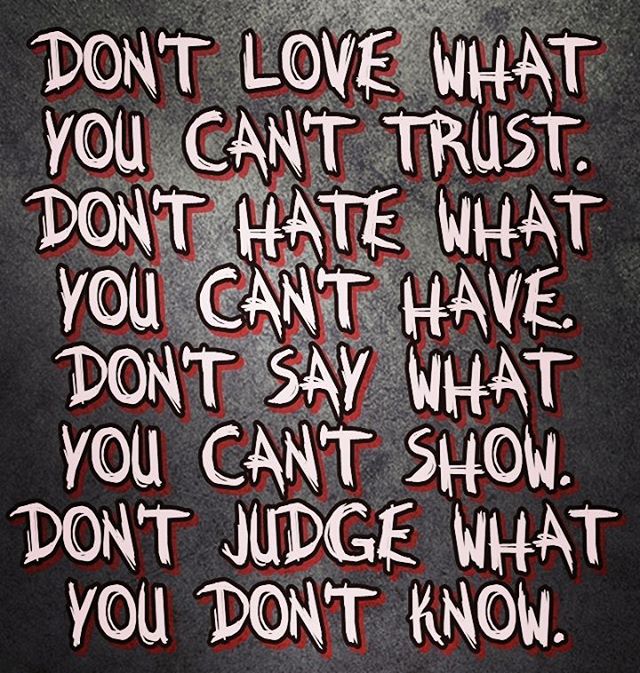The image appears to be a motivational quote flyer featuring the poignant message: "Don't love what you can't trust. Don't hate what you can't have. Don't say what you can't show. Don't judge what you don't know." The text is presented in a bold, freestyle font resembling paint strokes, with letters in white accented by red shadows and a black border, giving it a three-dimensional effect. The backdrop is a textured gray gradient that transitions from darker edges to a lighter center, mimicking the appearance of a chalkboard. The impactful message is visually organized into evenly spaced lines, each followed by a period, enhancing its readability and aesthetic appeal. This evocative design is typical of motivational pages that focus on delivering profound and reflective quotes.